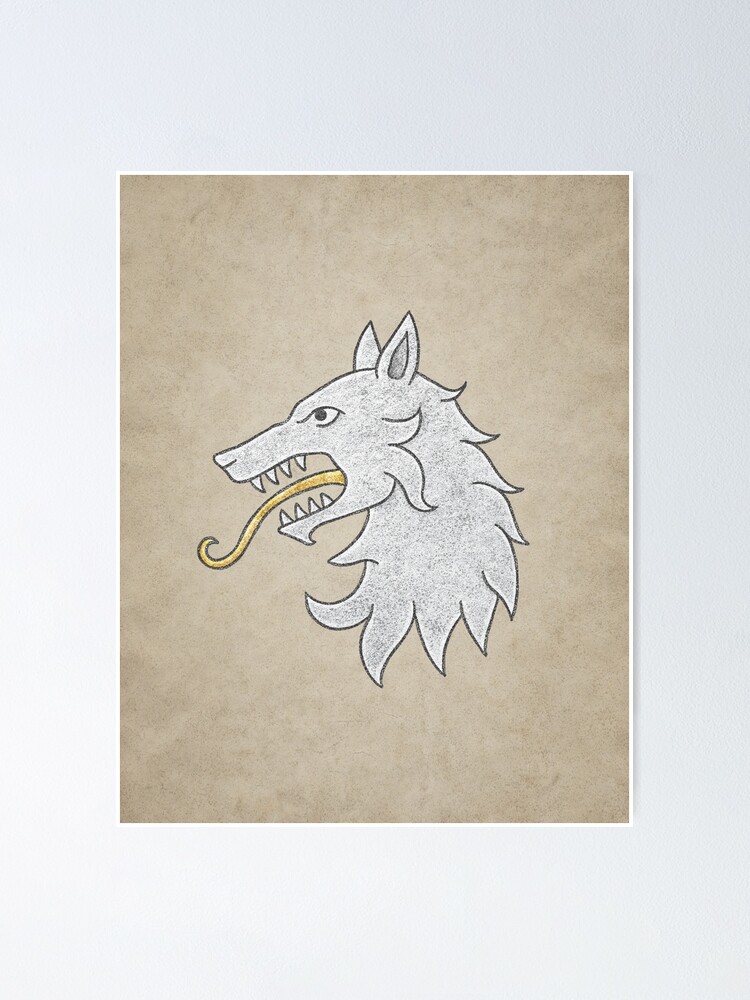A detailed pencil-drawn image of a wolf's head framed by a thin white border, set against a light gray-brown background with a gritty, paper bag-like texture. The wolf is depicted in left profile with its head facing left, displaying an angry expression emphasized by its perked ears, fierce black eye, and bared sharp teeth—four prominent ones on both the upper and lower jaws. The white fur of the wolf flows in wavy, spiky strands from its head down towards the bottom left of the image, accentuating the creature's intensity. Emerging from its gaping mouth is a strikingly long, curled yellow tongue, which twists into a hook-like shape at the end, adding a surreal touch to the otherwise realistic portrayal. The use of pencil and color suggests a detailed and carefully shaded technique, highlighting the wolf’s menacing demeanor.